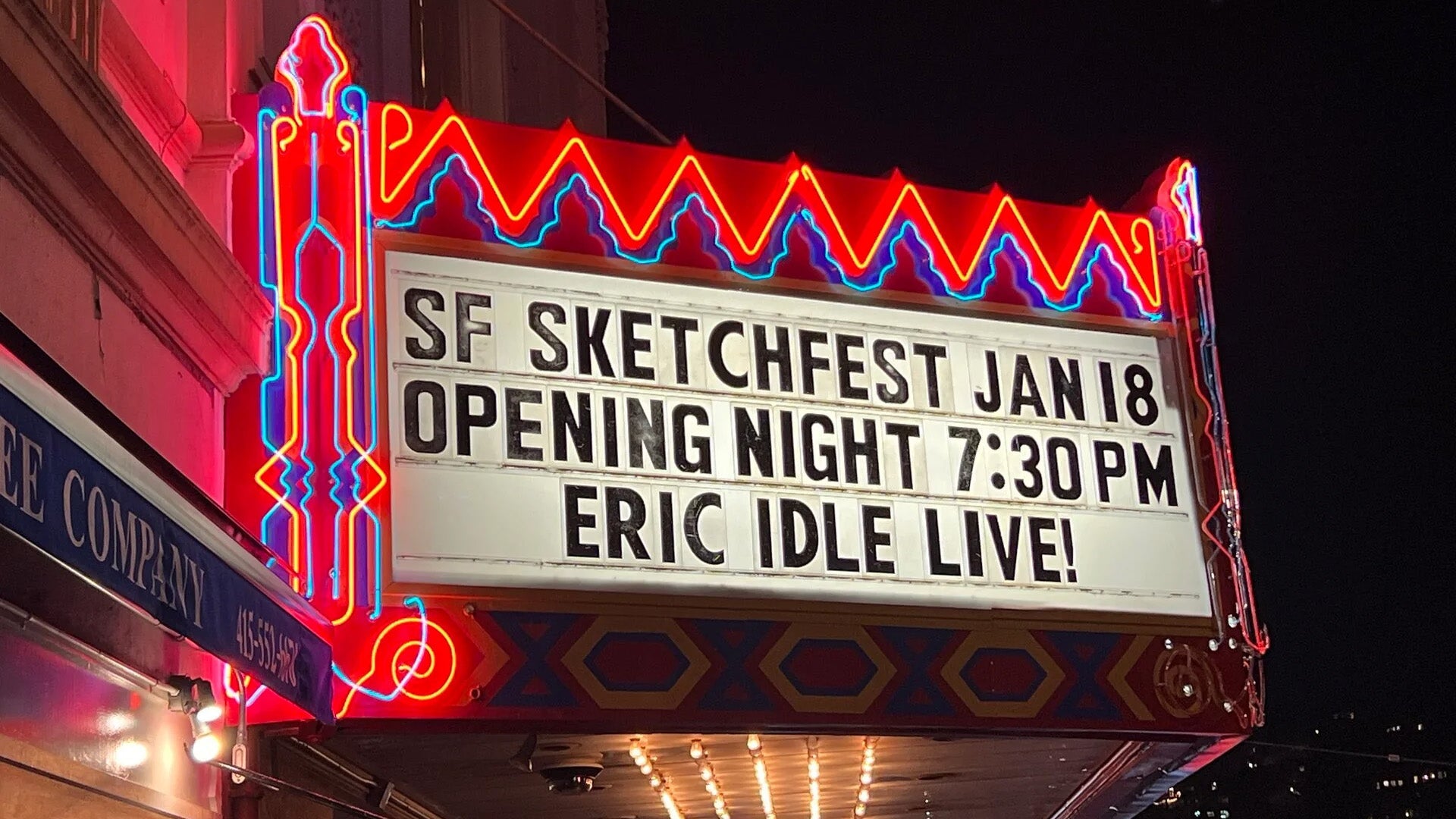The photograph captures the front entrance of a theater at night, showcasing a well-lit marquee with a black text on a white background. The marquee announces "SF SketchFest, January 18th, Opening Night, 7:30 PM, Eric Idle Live." The vibrant neon lights in orange, blue, and red form various shapes: a scepter on the left, mountain-like shapes at the top, and small octagonal lights along the bottom, making the sign stand out against the dark night sky. Additionally, there are lights adorning the theater's entrance roof. Another building is partially visible beside the theater, displaying The Something Company and a contact number, 415-552-667.